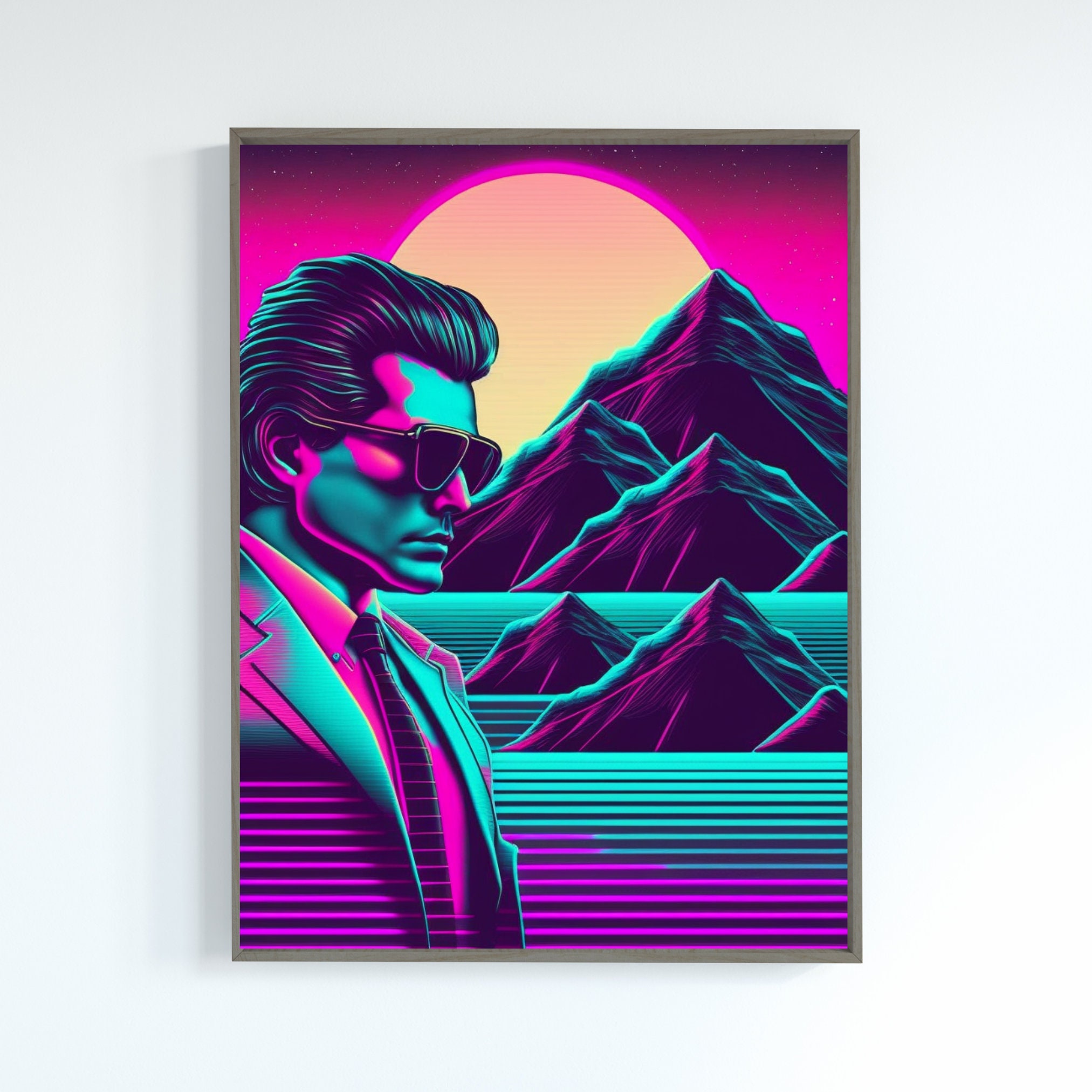This vibrant painting is a striking mix of neon hues, prominently featuring hot pink, green-blue, and purple shades. Shimmers abound throughout the piece. Dominating the composition is a large, radiant sun at the center, encircled by hot pink tones. The lower right section reveals a row of dark mountains accented with the same bright green-blue and hot pink colors, possibly mirrored in a body of water.

To the left, occupying about a third of the canvas, is the neutral-faced figure of a man in a suit. His white shirt is a vivid hot pink, complemented by a neon-striped tie that appears to depict shimmering waves. The man wears large sunglasses, with his short, dark hair slicked back. A blue line traverses the image, originating from the man and extending through the mountains, transitioning to different hues as it moves toward the bottom, ultimately shifting from blue to bright pink or purple. The overall contrast and dynamic colors make this artwork compelling and intricate.